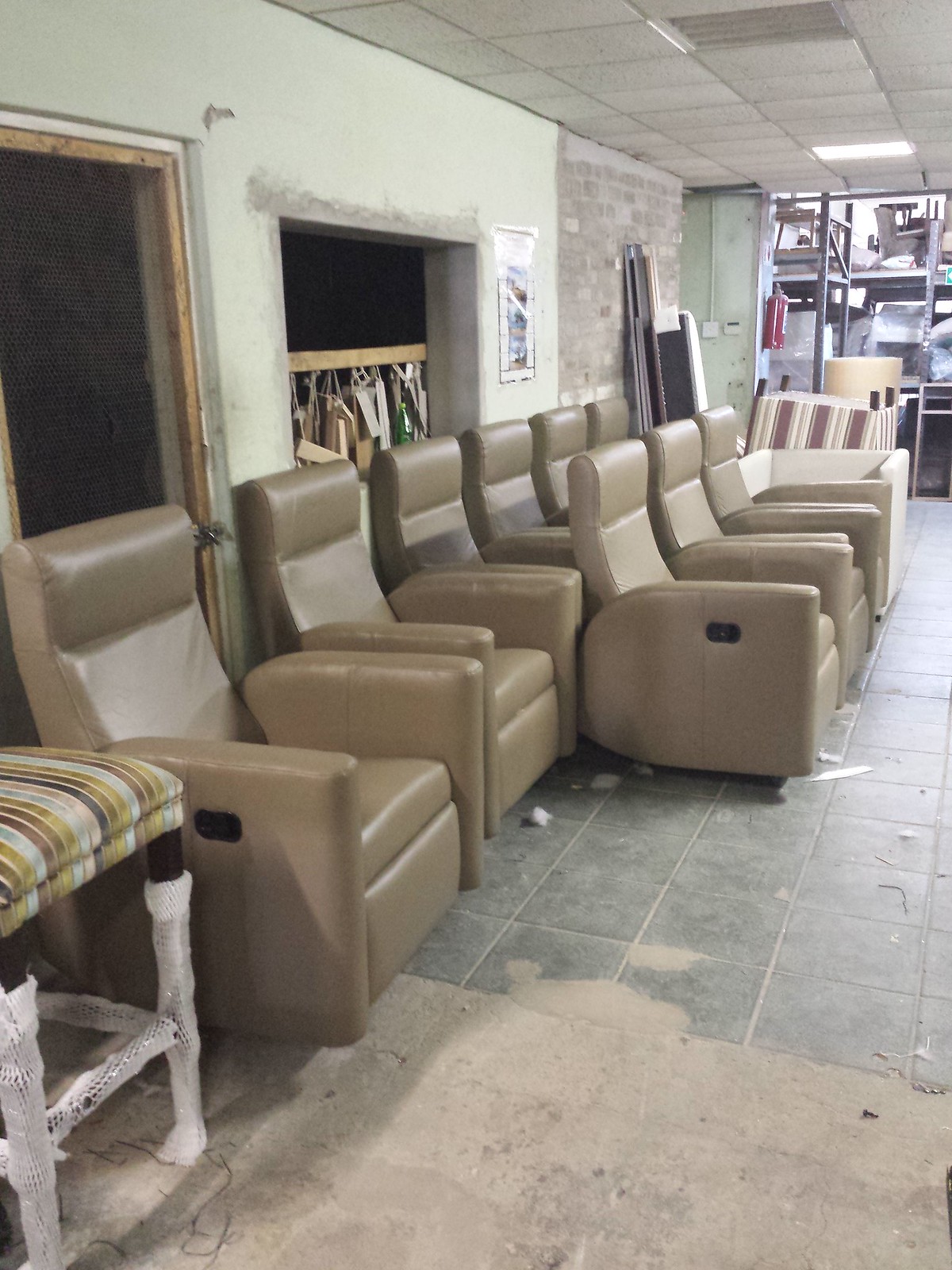In a worn and weathered storefront or office interior, an arrangement of nine beige leather recliners dominates the view, aligned in two rows. The back row, consisting of six recliners, stretches diagonally from the lower left-hand corner to the middle of the upper right quadrant, while the front row has three additional recliners placed directly in front of the last three in the back row. The recliners are firm, thin-armed, and equipped with black handles for footrests. The setting features a teal green wall marred by peeling paint and structural damage, interspersed with open window frames cut into squares. The floor, laid with cracked teal tiles, reveals patches of concrete underneath and shows significant signs of distress and age. A stool with frilly white legs and a striped cushion stands in the foreground at the bottom left. The left side of the image reveals an old coat hanger and a brick wall behind it, alongside a distant view through a window into an area filled with various chairs, desks, and furniture. In the upper right background, three shelf units bear miscellaneous items, contributing to the overall sense of clutter.